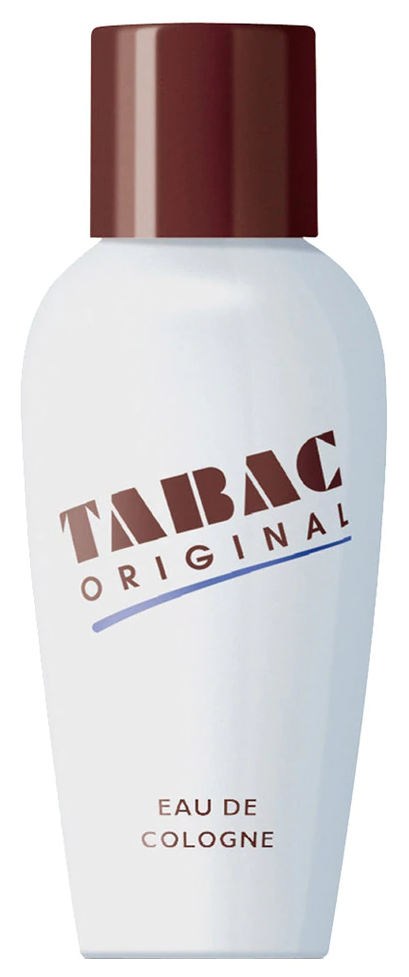This photograph features a distinctive bottle of eau de cologne. The bottle is white, presenting a short and squat silhouette that commands attention. Topping the bottle is an oversized brown cap, which adds a touch of elegance and balance to its stature. The bottle's label is adorned with bold, thick block lettering arranged diagonally, spelling out "T-A-B-A-C." Below this, the word "Originals" is printed in a less prominent block lettering, accentuated by a blue stripe underlining it. Along the lower portion of the bottle, the phrase "Eau de Cologne" appears in smaller, yet still compelling, brown block lettering. The intricate play of typography and color on the minimalist white bottle creates a tasteful and refined appearance.